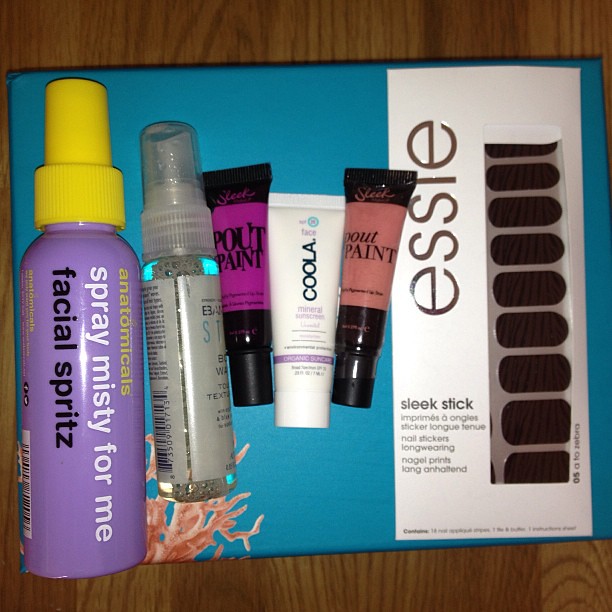This photograph showcases an assortment of beauty and health products meticulously arranged atop a dual-colored box on a dark reddish-brown wooden table. The box itself features a blue left side and a white rectangle on the right, with vertically aligned text reading "Essie." In the foreground, the text "Sleek Stick" is visible, though the font below is too small to decipher.

Starting from the left, there is a prominent purple bottle with a yellow lid labeled "Spray Misty For Me" in white font, and "Facial Spritz" in black font beneath it. Next to it, there's a gray bottle with a sparkly clear lid, presenting an elegant touch. The middle of the lineup features a black squeeze bottle with a pink label marked "Pout Paint." Following that is a smaller white squeeze bottle labeled "Mineral Sunscreen Face Coola." On the far right, there is another black squeeze bottle, this one adorned with an orange or reddish-brown label, also identified as "Pout Paint." In addition to these bottles, there's a flat paper item resting on the box, contributing to the detailed composition of the scene.